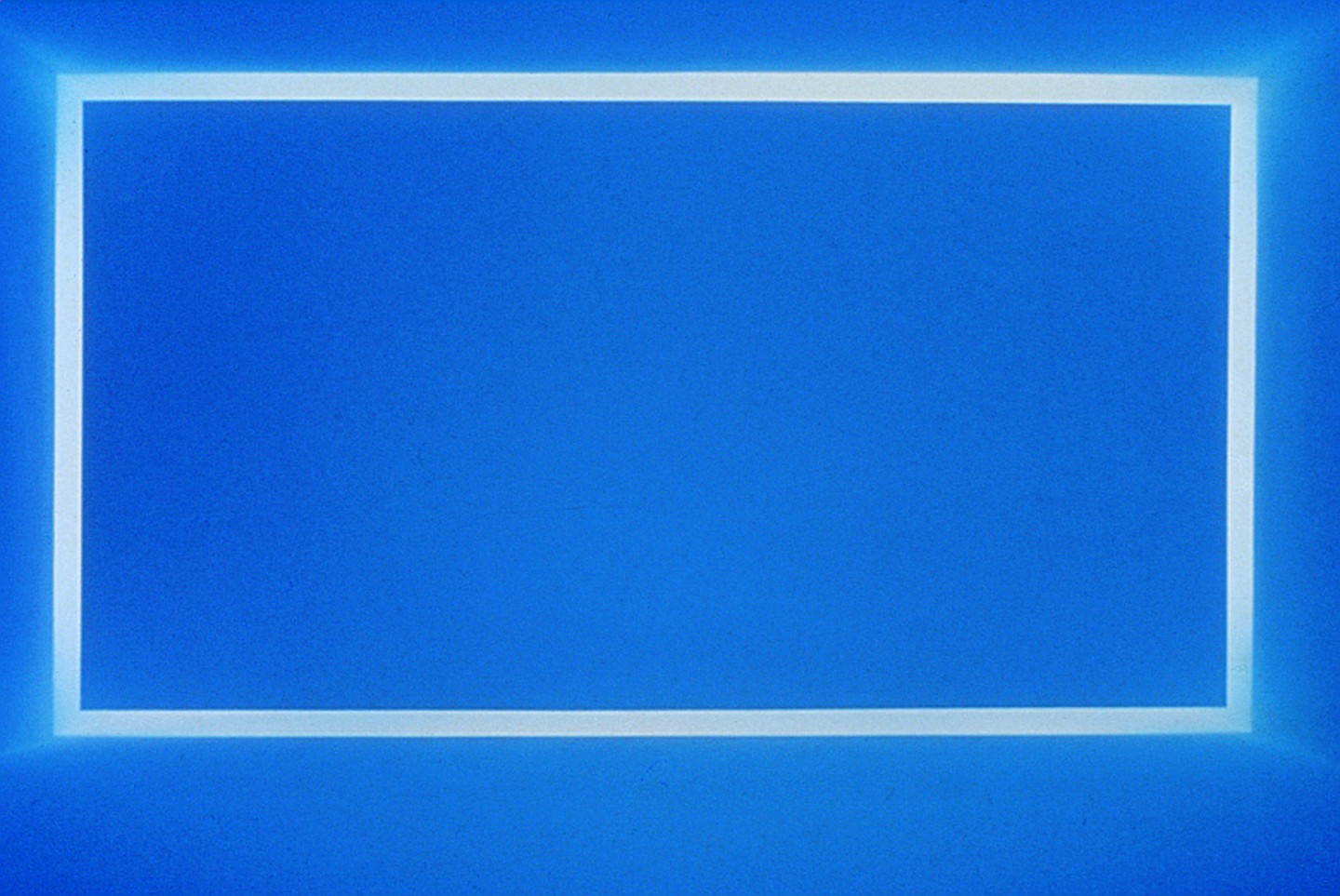The image is horizontally framed and dominated by a striking royal blue background. Centrally positioned, though slightly higher than the middle, is a thin, silver rectangle resembling the shape of a widescreen television or movie theater screen, occupying approximately two-thirds to three-fourths of the entire frame. This rectangle is characterized by its delicate, shining silver borders, reflecting a subtle white light that contrasts against the intense blue backdrop. The blue color of the image is the most prominent feature, with the silver rectangle adding an intriguing focal point to the composition.